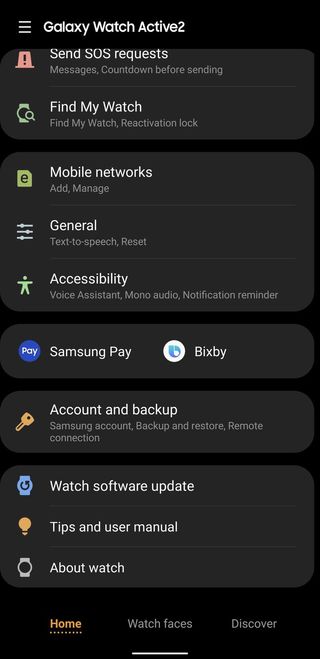The image displays the settings menu of the Galaxy Watch Active 2 within its companion app on a smartphone. At the top, it highlights the watch model, "Galaxy Watch Active 2." This comprehensive menu allows users to manage various settings of the watch directly from their phone. Key features of the menu include an option to send SOS requests and messages with a countdown timer, a "Find My Watch" function likely utilizing GPS and possibly emitting sound to locate the device, and the ability to lock the watch if it gets lost or stolen.

Further down, the menu offers settings for mobile networks, general settings, and accessibility. Dedicated buttons for Samsung Pay and Bixby are also present, alongside options for account management and backup, ensuring users can secure their data and account details. The "Watch Software Updates" option provides a way to update the watch's software. Additionally, the menu includes a "Tips and User Manual" section for user guidance, and an "About Watch" section that details the current software version and other pertinent information about the watch.